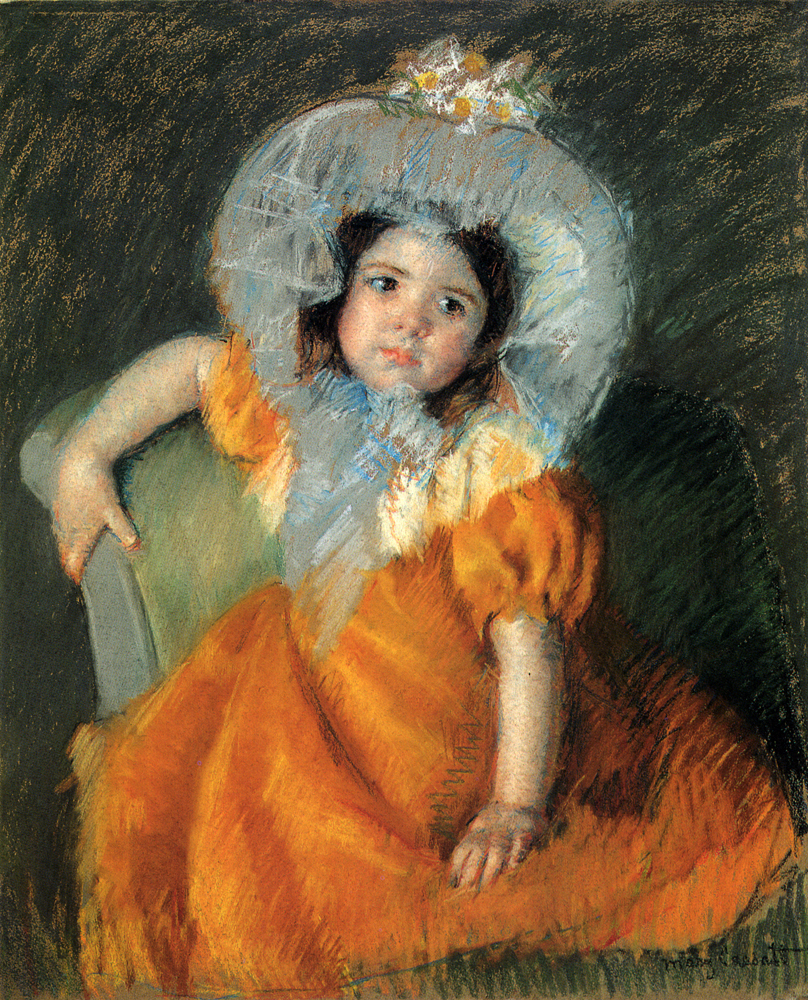The painting is an oil portrait of a young girl, aged between 5 and 10 years old, with brown hair and soft brown eyes. She is wearing a vibrant orange dress with puffy cap sleeves and a white headdress adorned with a large blue bonnet tied under her chin. This bonnet is decorated with white and yellow flowers at its center and sits atop her head like a halo, additionally accented by a white bow. The girl's expression is soft, with peach-colored lips and a slightly sad, or perhaps confused, demeanor as she looks off to the left. She is seated on a green chair; her right hand rests on its back while her left hand gently rests on her lap. The background is a deep green with varied brushstrokes, creating a faded effect that contrasts subtly with the vividness of her attire. The painting is signed in the bottom right corner, though the name is not easily discernible.